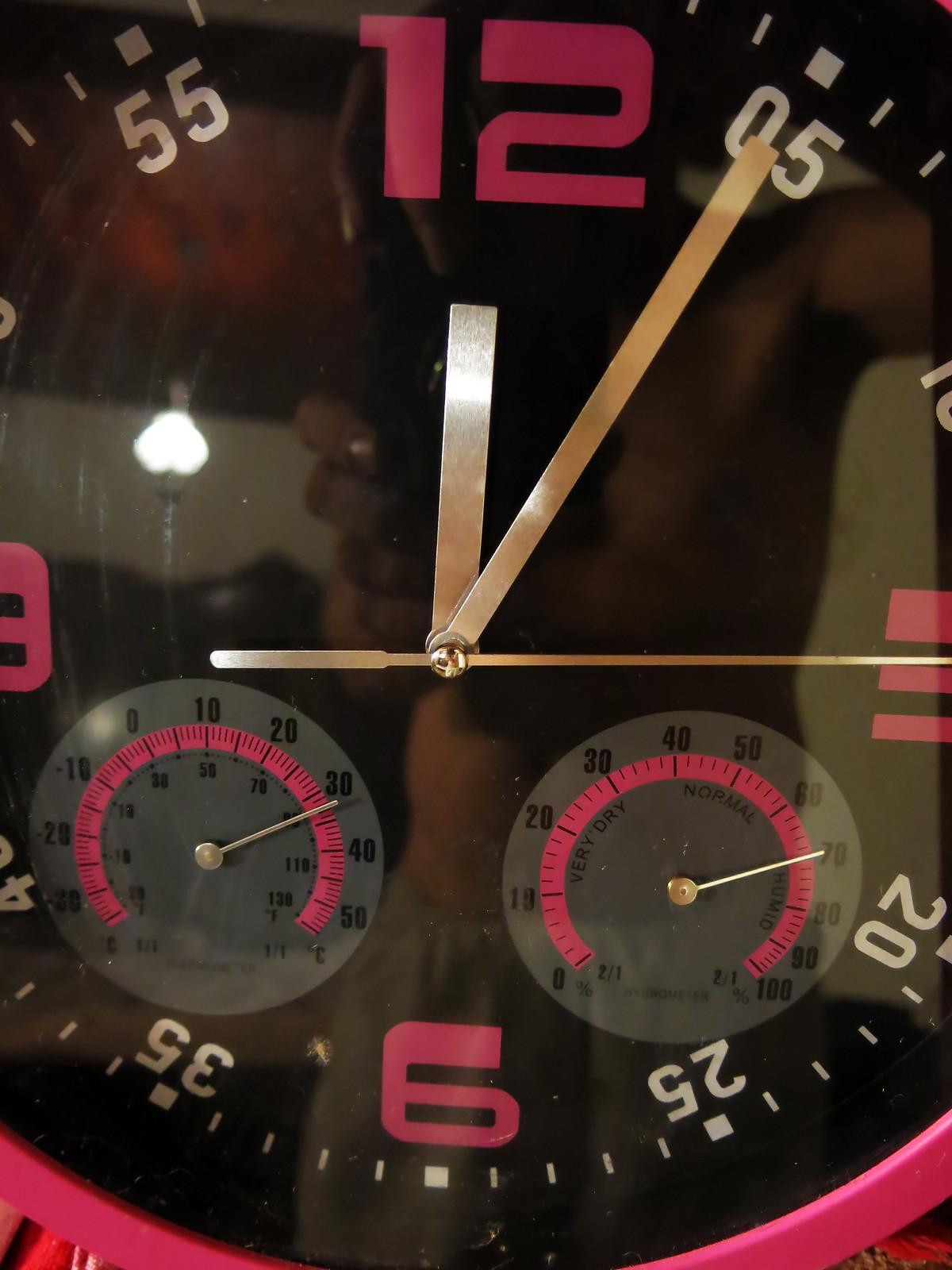This close-up photograph captures a unique and vibrant clock with an intriguing design. The clock's face stands out against a solid black background, making the vibrant colors and intricate details pop. The main hour markers—12, 3, 6, and 9—are brightly highlighted in fluorescent pink, while the remaining numerals, including 1, 2, 4, 5, 7, 8, 10, and 11, are in contrasting white. This creates a striking visual effect that draws the viewer in. The clock hands—comprising the hour, minute, and second hands—are fashioned from sleek stainless steel, adding a touch of modern elegance.

Adding to the clock's uniqueness are two auxiliary dials embedded within the main face. One of these dials appears to measure a range from 0 to 100, likely indicating humidity levels in percentage form. The second dial measures temperature, spanning from -30 to 50 degrees Celsius, thus providing an additional layer of functionality. This clock intertwines practicality with a bold, avant-garde aesthetic, making it a fascinating centerpiece.